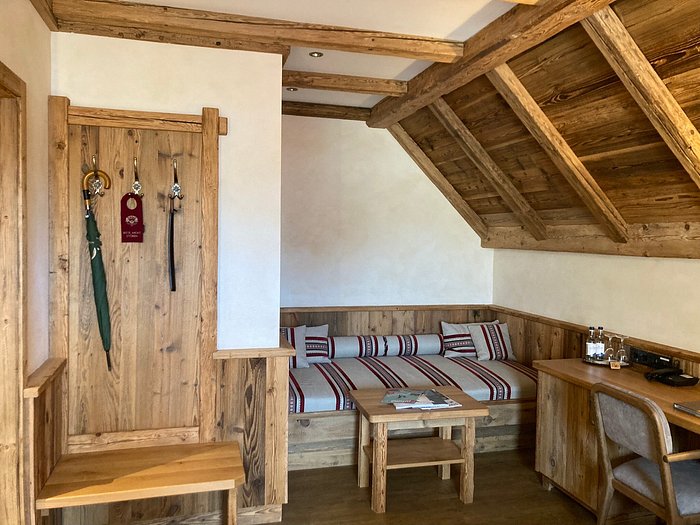This image depicts a cozy, multi-functional room that blends elements of a bedroom and working space, with a strong wooden aesthetic. The room, which might be part of a house, cabin, or possibly a hotel, features various wooden elements, creating a warm, rustic atmosphere. On the left-hand side, there is a wooden door or an elevated closet with an umbrella, a shoe horn, and a placard hanging from it. Below this, a wooden bench provides a spot to sit and remove shoes. Adjacent to this, a built-in nook with a low and wide cushioned seat, adorned in white fabric with red stripes, functions as both a seating area and a potential sleeping space. A small table sits in front of this nook. To the right, a desk accompanied by a chair adds a workspace element to the room. The walls are white with wooden borders along the bottom half, and the ceiling features a unique angled wooden section that slopes from the wall to the roof, adding to the cabin-like charm. Some items are placed on the table, although their specifics are unclear.